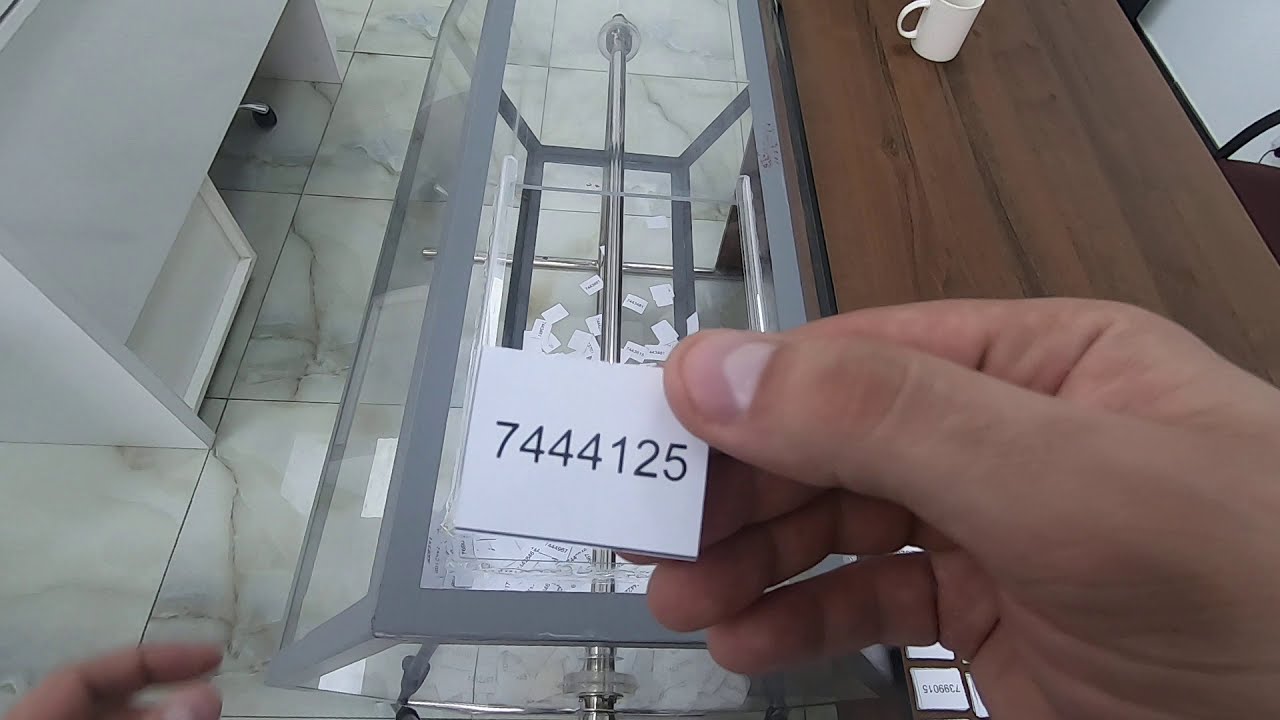The color photograph captures an indoor scene viewed from above in a landscape orientation, showcasing a meticulously detailed and realistic environment. Centered prominently in the image, a hand emerging from the right side holds a small white slip of paper with the numbers "R7444125" printed in bold black text. A portion of another hand, slightly blurred, is visible on the left edge of the frame, hinting at a secondary presence.

The background features a sophisticated array of items and surfaces: directly underneath the slip of paper is a glass tabletop supported by a silver bar, which appears to be part of a larger contraption made of glass and gray metal, filled with similar-numbered slips. To the right, a large brown wooden table stands, adorned with a white mug positioned near the top edge of the image. On the left side, part of a white desk or piece of furniture is visible. The scene is set against a backdrop of polished white marble flooring veined with gray streaks, enhancing the overall refined and modern aesthetic.